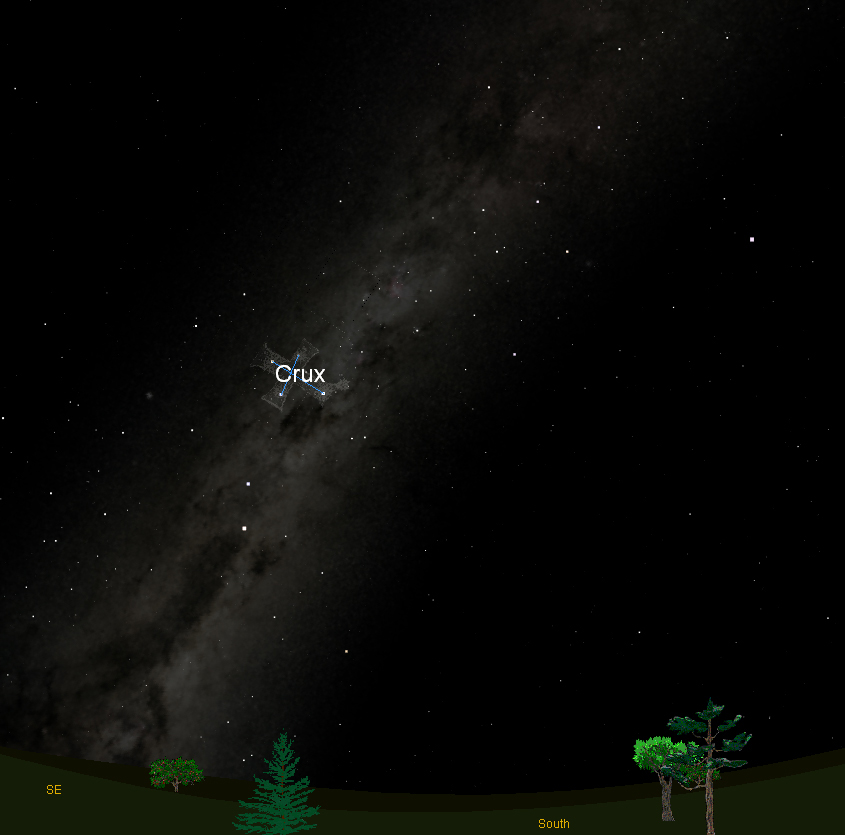This is a digital drawing resembling a scene created with basic graphics software like Microsoft Paint or clip art. The sky is pitch black with scattered white stars, forming a clear portrayal of a night scene. In the middle of the sky, a constellation named Crux ( C-R-U-X ) is prominently marked with blue lines connecting its stars, highlighting its cross shape. The constellation is the only one labeled in the image. Stars are primarily arranged in a diagonal formation, running from the lower left to the upper right corner. Below the sky, there is an olive green, rolling field featuring a few pixelated trees, including a pine tree and an apple tree with little red dots representing apples. Off to the sides, additional trees appear to be an oak and other mixed species. The bottom of the image contains text with the words “South” and “SE” (Southeast) written in yellow. There is also a small, less discernible section of dark gray splotches, possibly representing a Milky Way-like pattern, accentuating the nighttime vibe. The image is simple yet detailed, capturing the serene essence of a starry night.